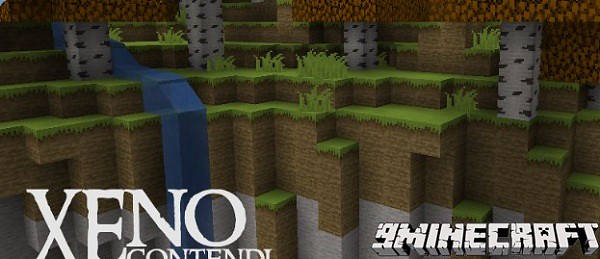A detailed and descriptive caption for the image could be:

"An up-close view of a Minecraft scene showcases multiple terraces in the background, each adorned with lush green grass and a variety of plants. The terraces are layered, providing depth to the landscape, and feature a striking blue waterfall cascading down the left side. Among the vegetation, several birch trees stand out with their distinctive white bark and black splotches, their branches adorned with vibrant leaves. Although minimal activity is present, the scene suggests it could be from the opening sequence of the game, highlighted by elements like the number '9' associated with Minecraft."